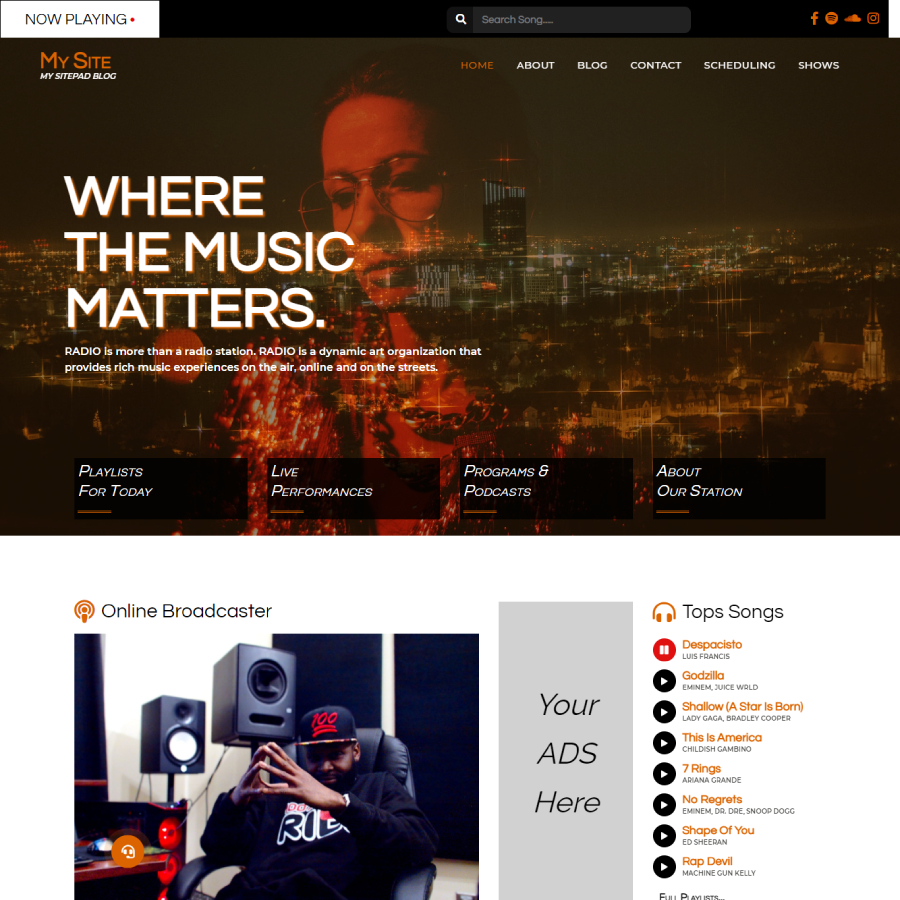This image depicts a website titled "My Site Pad Blog" characterized by a white, black, and orange color scheme. The logo "My Site" is written in orange text, with "My Site Pad Blog" in white text directly beneath it. Above the logo, there is a "Now Playing" indicator in white text, accompanied by a red live dot symbolizing live content. 

At the top of the webpage, a search bar labeled "Search Song" is featured prominently. To the right of this bar, there are orange-colored icons linked to social media platforms, including Facebook, Spotify, SoundCloud, and Instagram, serving as contact information.

The banner image at the top showcases a monochromatic orange-tinted nighttime skyline, highlighting various buildings and residential areas illuminated by city lights. Overlaying this cityscape is an image of a woman wearing glasses, looking contemplatively. Above the image, the slogan "Where the Music Matters" is displayed. 

Below this banner, there is a tagline that reads: "Radio is more than a radio station. Radio is a dynamic art organization that provides rich music experiences on the air, online, and on the streets."

The navigation menu at the top of the website includes tabs labeled Home, About, Blog, Contact, Scheduling, and Show, with the Home tab highlighted in orange to indicate its selection.

Further down the page, there are various sections including tabs for additional information and what appears to be curated playlists, along with an advertisement space labeled "Your Ad's Here". Additionally, there is an ad displaying "Online Broadcaster," featuring an image of a man in a studio with his fingers steepled, promoting some sort of template for advertisers.